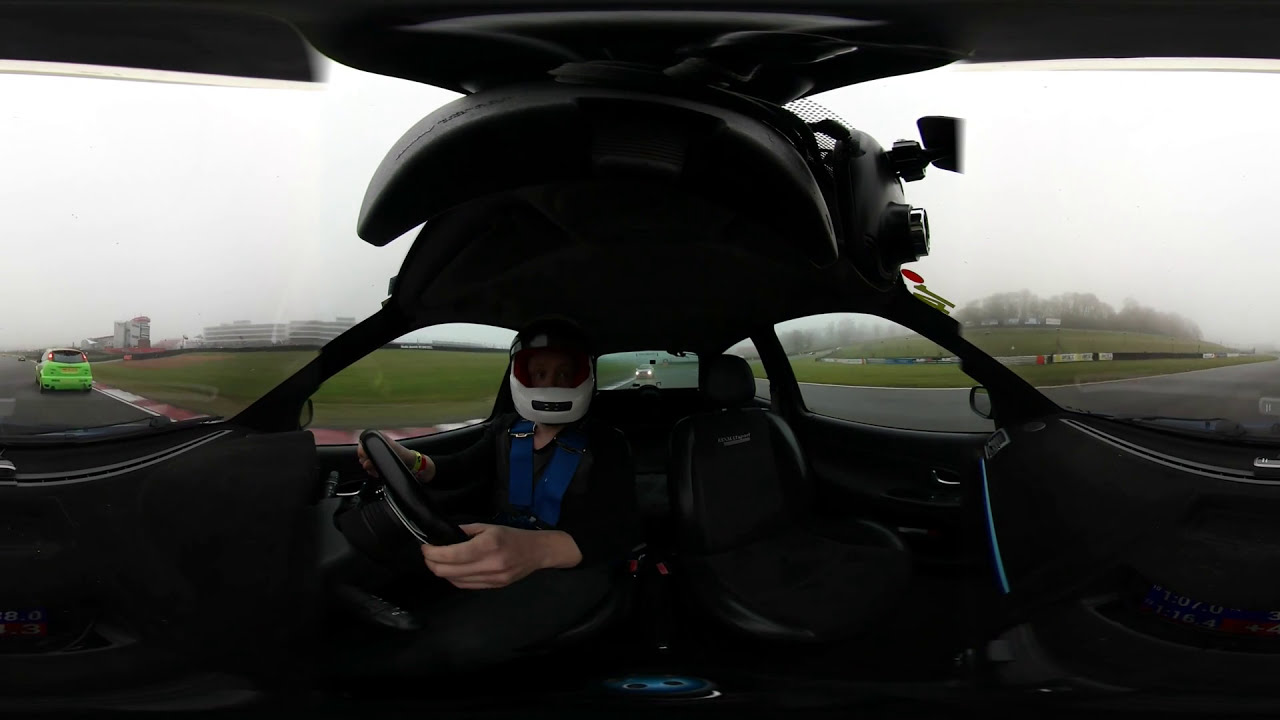The image depicts an individual, possibly a woman, wearing a white helmet with a mask, seated in a race car. The person, identifiable only by their eyes and tan hands adorned with yellow and red bracelets, grips a black steering wheel inside a sleek, black interior of what appears to be a specialized sports vehicle. The setting is a race track characterized by alternating red and white racing lines on the left, grassy expanses, and a fence adorned with advertisements. Surrounding the track are several vehicles, including a green minivan with red lights ahead and a white or gray car with headlights on behind. The sky is overcast and hazy, suggesting an imminent rain. The scene is framed by nearby structures and additional tracks, all contributing to the bustling and competitive atmosphere of the race track.